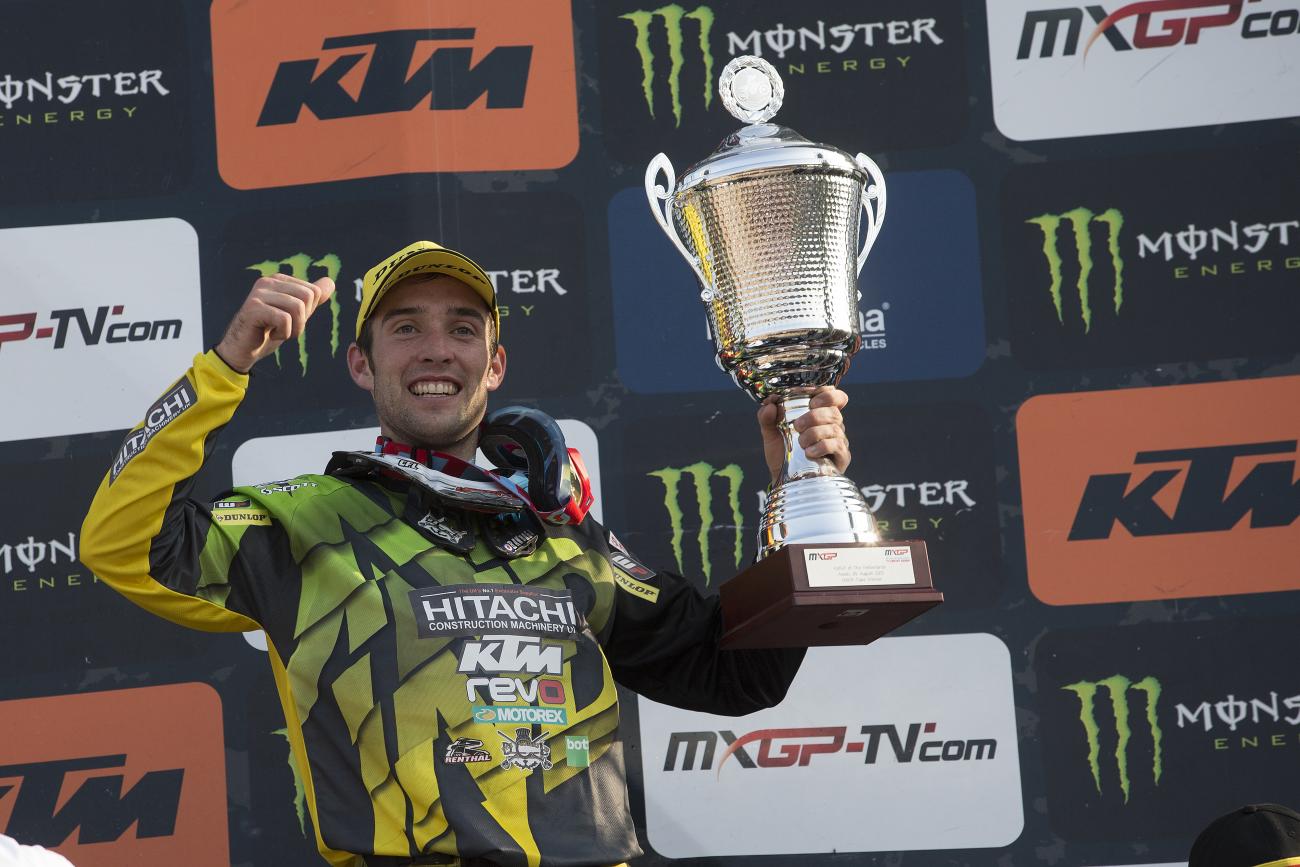In this detailed image, a jubilant man, decked out in striking racing gear, stands proudly before a backdrop filled with diverse sponsor advertisements, including Monster Energy, KTM, and MXGPTV.com. His outfit is a vibrant blend of black, lighter green, and bright yellow, with the name "Itachi" prominently displayed. A helmet complements his racing attire, signifying his recent participation in a high-stakes race. The sponsorship-laden banner behind him further highlights the event's competitive nature, featuring logos like KTM and Monster, as well as unclear ones such as KTLM and NM KTLM. Clutching a large trophy, the man visibly celebrates his victory, his excitement palpable, suggesting a significant achievement, possibly within a competitive racing league, perhaps NASCAR. The entire scene is a whirlwind of colors and emotions, highlighted by his conspicuous yellow vest and hat, against a backdrop of black, white, red, green, and yellow elements.